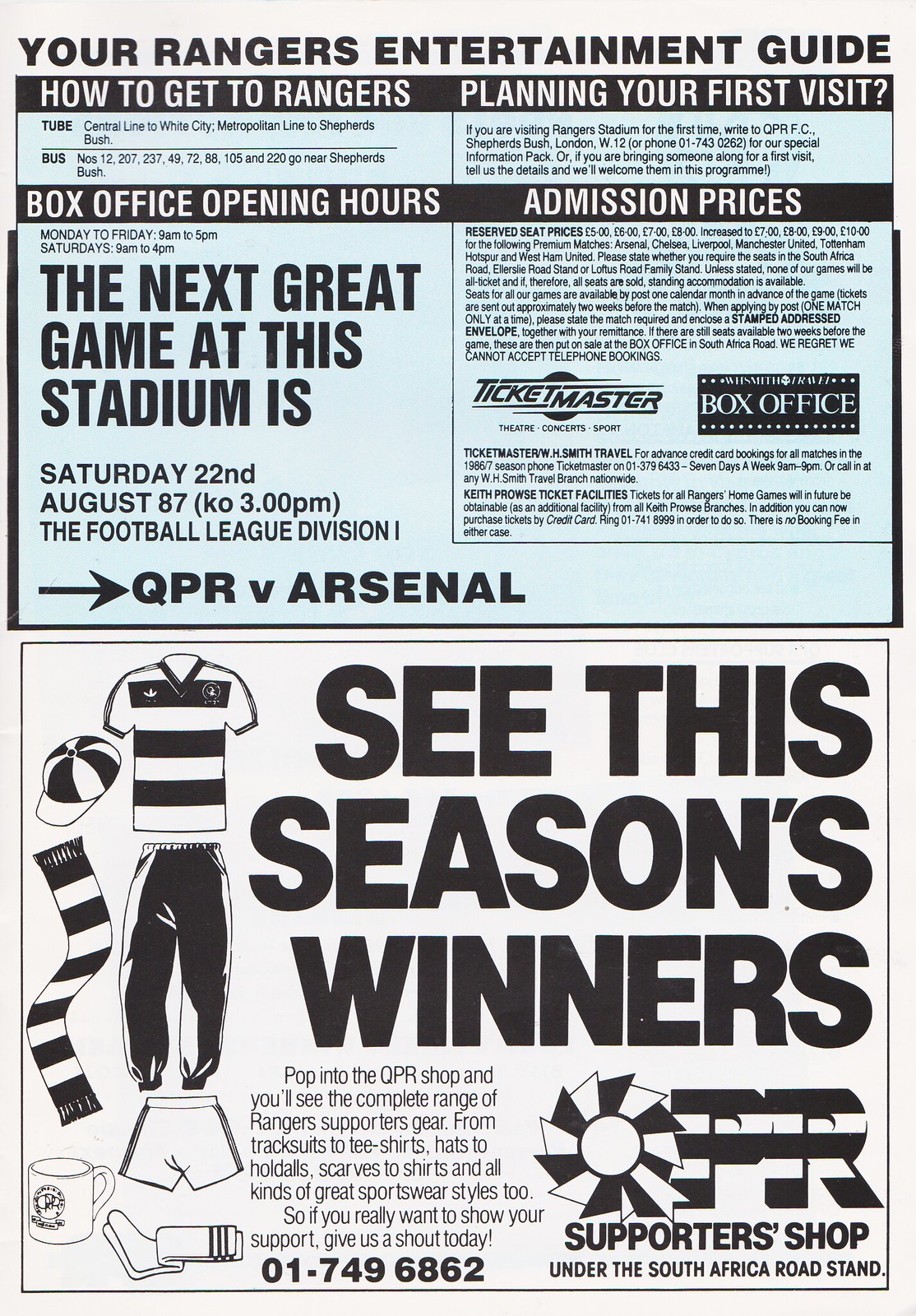This image depicts a vintage black-and-white print publication, specifically an athletic program guide with spot color elements. The publication is designed in portrait orientation and prominently features "Your Rangers Entertainment Guide" in black, all-caps text at the top. Below this headline is a comprehensive half-page advertisement detailing information about obtaining Rangers tickets, box office opening hours, and specifics about the next big game, scheduled for Saturday, 22nd August 1987, with QPR facing Arsenal. Ticket prices and instructions for booking, including premium matches against teams like Arsenal, Chelsea, Liverpool, Manchester United, Tottenham Hotspur, and West Ham United, are also presented.

The bottom half of the page emphasizes the QPR Supporters Shop, located under the South Africa Road Stand. A bold headline states, "See this season's winners." Accompanying the text are black-and-white line drawings of various items available at the shop, including a shirt, cap, pants, shorts, socks, scarf, and a mug. There is an invitation to explore the full range of Rangers supporters' gear, from tracksuits to t-shirts and hats to scarves, encouraging fans to show their support. Additionally, detailed contact information is provided, including a phone number in bold fonts for further inquiries. The section is decorated with a PR/QPR logo and the descriptive tagline "Supporters Shop under the South Africa Road Stand" at the bottom right.